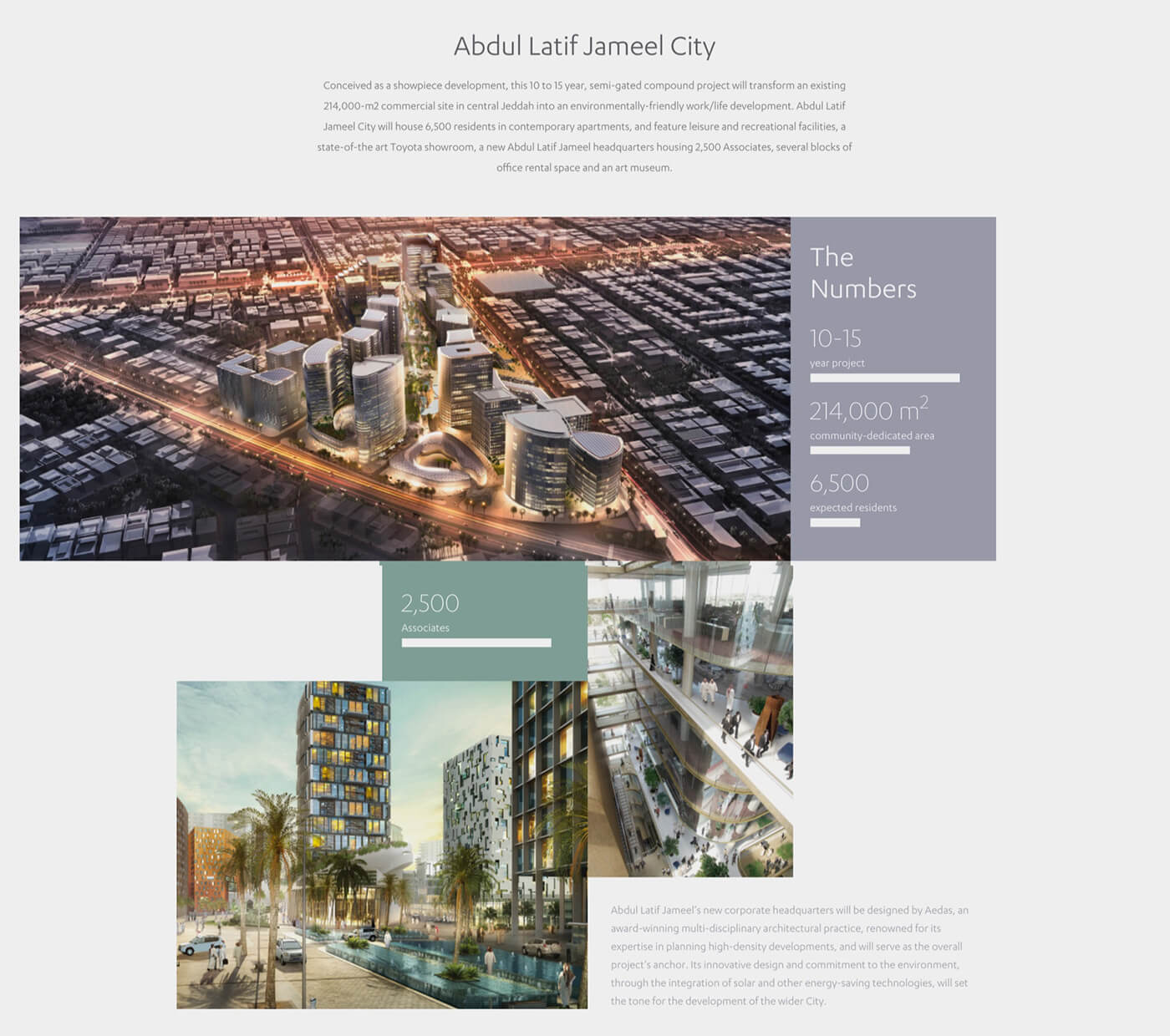The image features the official website for Abdul Latif Jameel City. At the top center of the image, the website's background is a light gray color. Prominently displayed is the name "Abdul Latif Jameel City," followed by a detailed description: "Conceived as a showpiece development, this 10 to 15-year semi-gated compound project will transform an existing 214,000 square meter commercial site in central Jeddah into an environmentally friendly work-life development." The text elaborates that Abdul Latif Jameel City will accommodate 6,500 residents in modern apartments and include leisure and recreational facilities, a state-of-the-art Toyota showroom, a new headquarters for Abdul Latif Jameel employing 2,500 associates, multiple blocks of office rental space, and an art museum. Below this text is an image of the city, along with a reference to the project's timeline of 10 to 15 years.